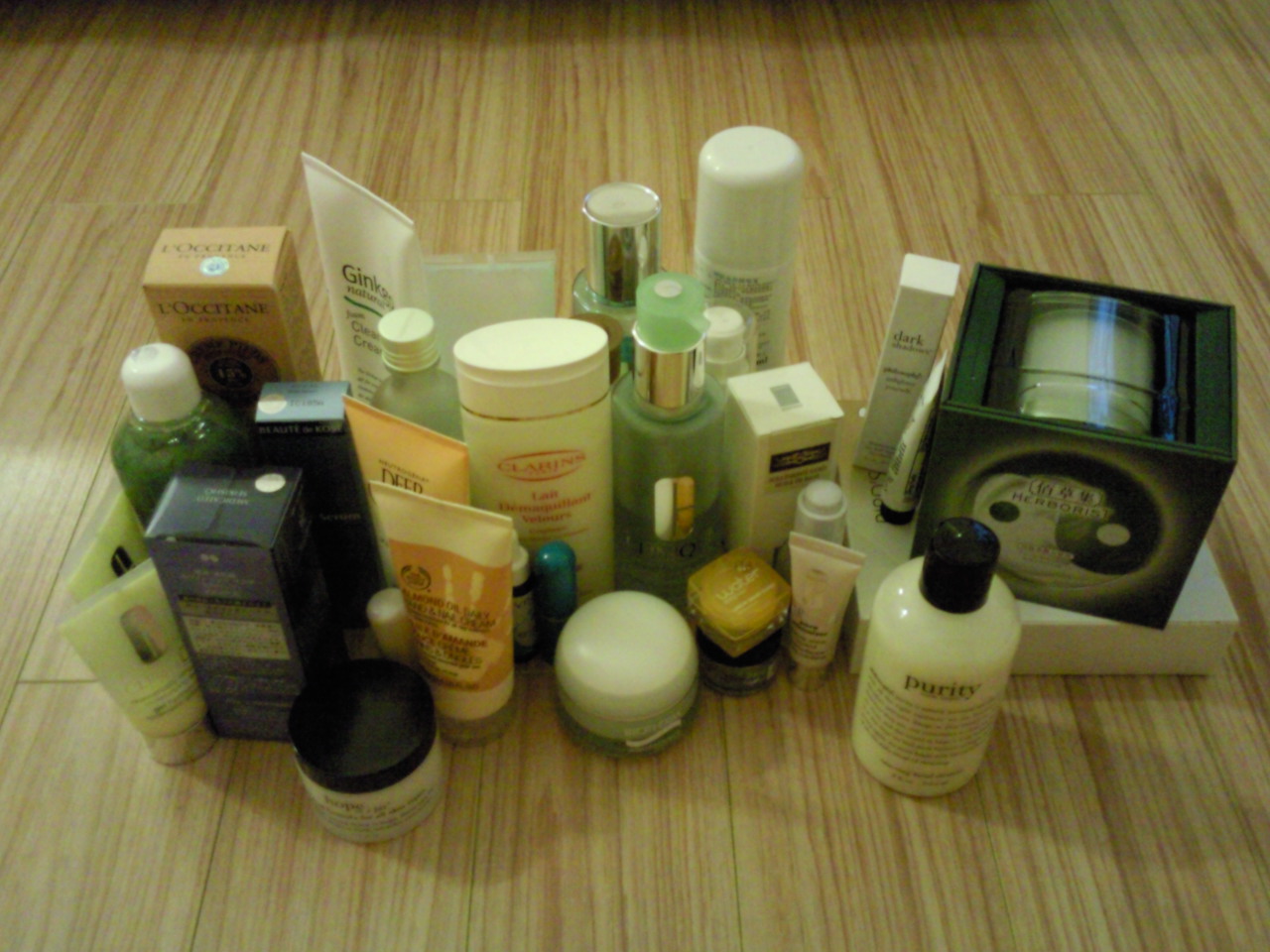On a light wood-colored table is an assorted collection of cosmetics, displaying an array of bottles, jars, and tubes in various shapes and sizes. Dominating the foreground is a white bottle labeled "Purity," distinguished by its black lettering and matching black cap. Scattered across the table are numerous containers, some tall, some small, each carrying cosmetic products. A Clinique tube is notably visible among the items, with another Clinique product discernible in the background. Towards the back, a L'Occitane box stands out amidst the mix.

The scene is filled with mostly muted colors, featuring greens, browns, whites, blacks, golds, and yellows, contributing to a calm, sophisticated palette. Beyond the containers, there is a neatly wrapped bar of soap, placed on a holder, hinting at luxury skincare. The collection encompasses a variety of items, including lipsticks, face creams, and body creams, presenting a comprehensive snapshot of a well-stocked cosmetic assortment on a wooden table.